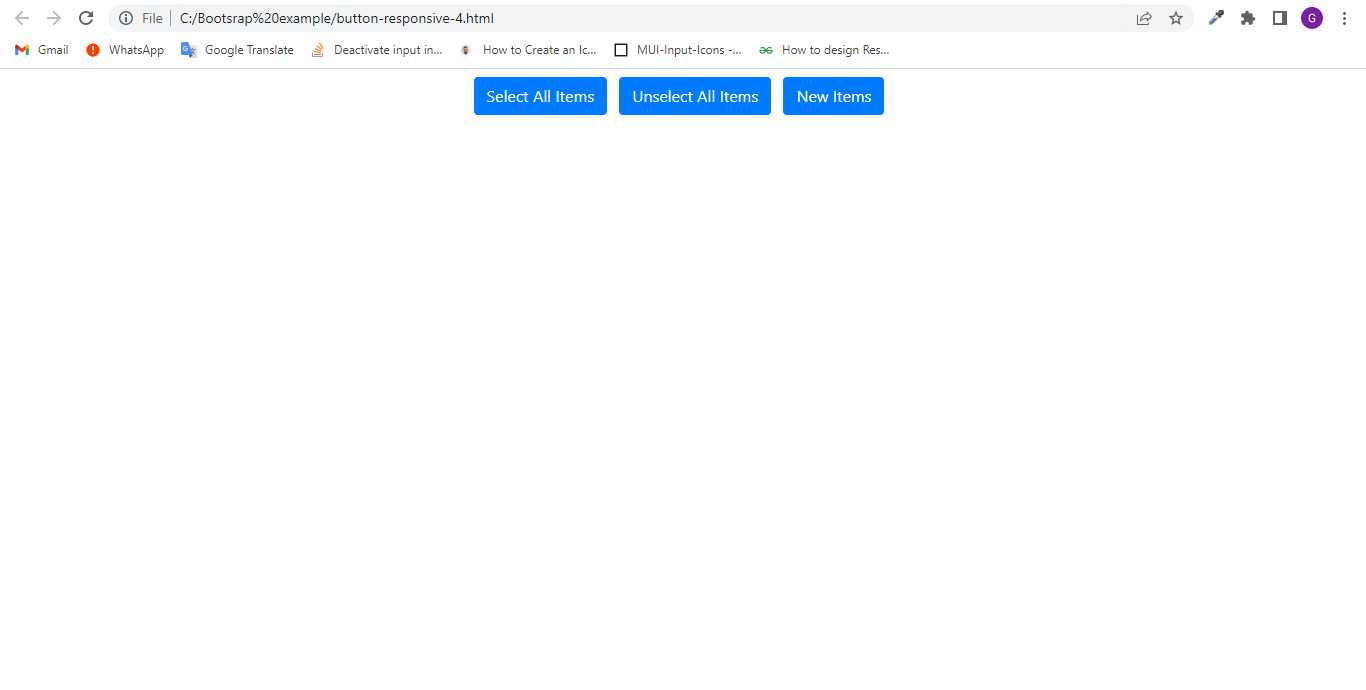The webpage depicted in the image features a web address bar at the top, displaying the URL: "c:/bootstrap%20example/button-responsive-4.html". Below the address bar, there are several saved icons representing options such as Gmail, WhatsApp, Google Translate, "Deactivate Input for Something", "How to Create Something", "MUI-Input Icons", and "How to Design Something".

Beneath these icons, there are three prominent, bright blue buttons arranged horizontally. The buttons are: "Select All Items", "Unselect All Items", and "New Items". Each button is rectangular with white text clearly indicating its function.

The rest of the webpage remains completely empty, set against a clean, white background.